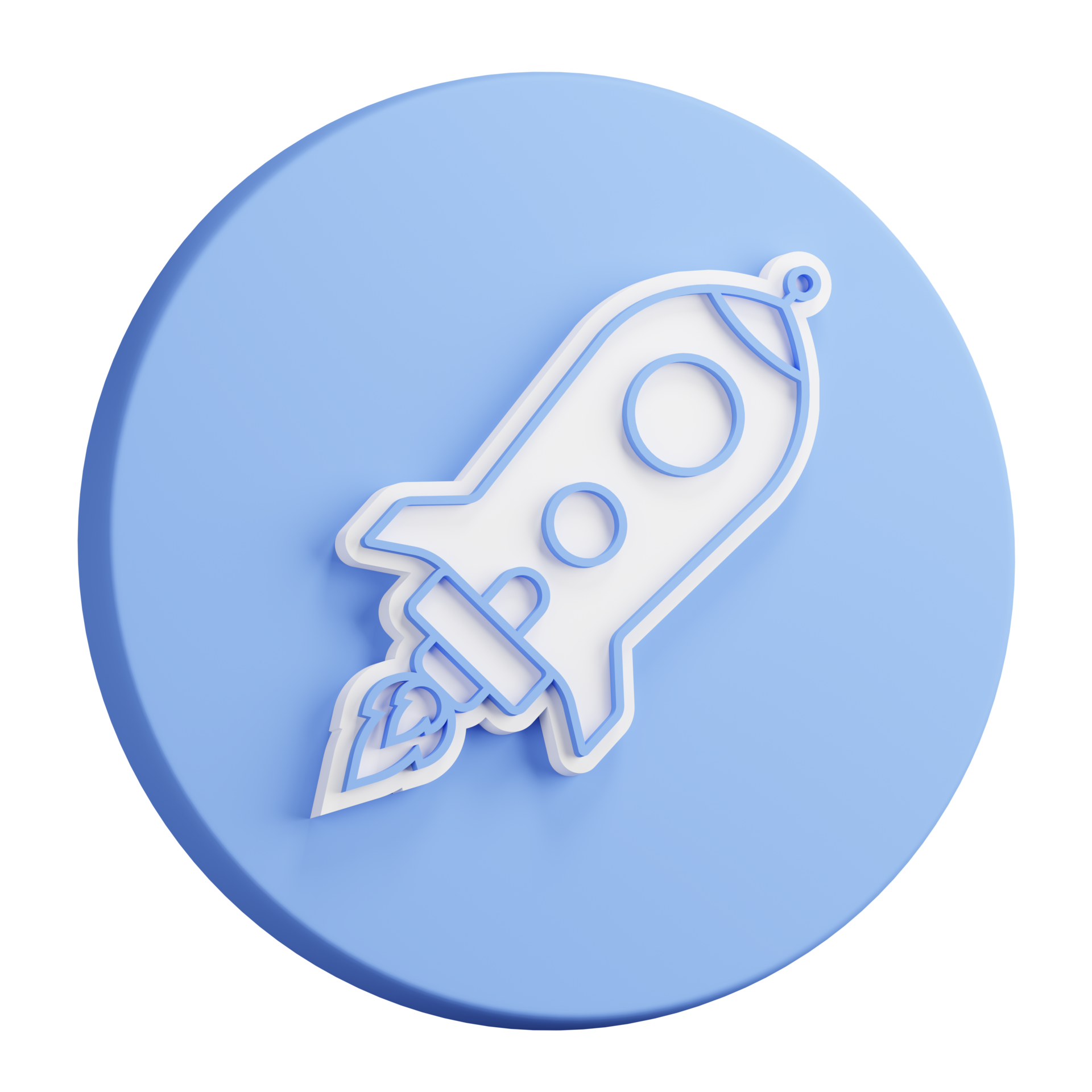The image depicts a minimalistic, close-up logo set against a stark black background. Dominating the scene is a circular, flat, 2D shape in a solid light blue color with a darker blue border along the top, left, and bottom edges. Centrally positioned within this circle is a white rocket ship, outlined with the same light blue hue of the circle. The rocket is tilted approximately 45 degrees clockwise. Detailed features include a small loop at the rocket's top, two circular windows at its center, and blue flame-like elements emerging from its base, which hints at motion. The simplicity of the design is highlighted by its clean, uncluttered presentation and the absence of any additional objects or text.